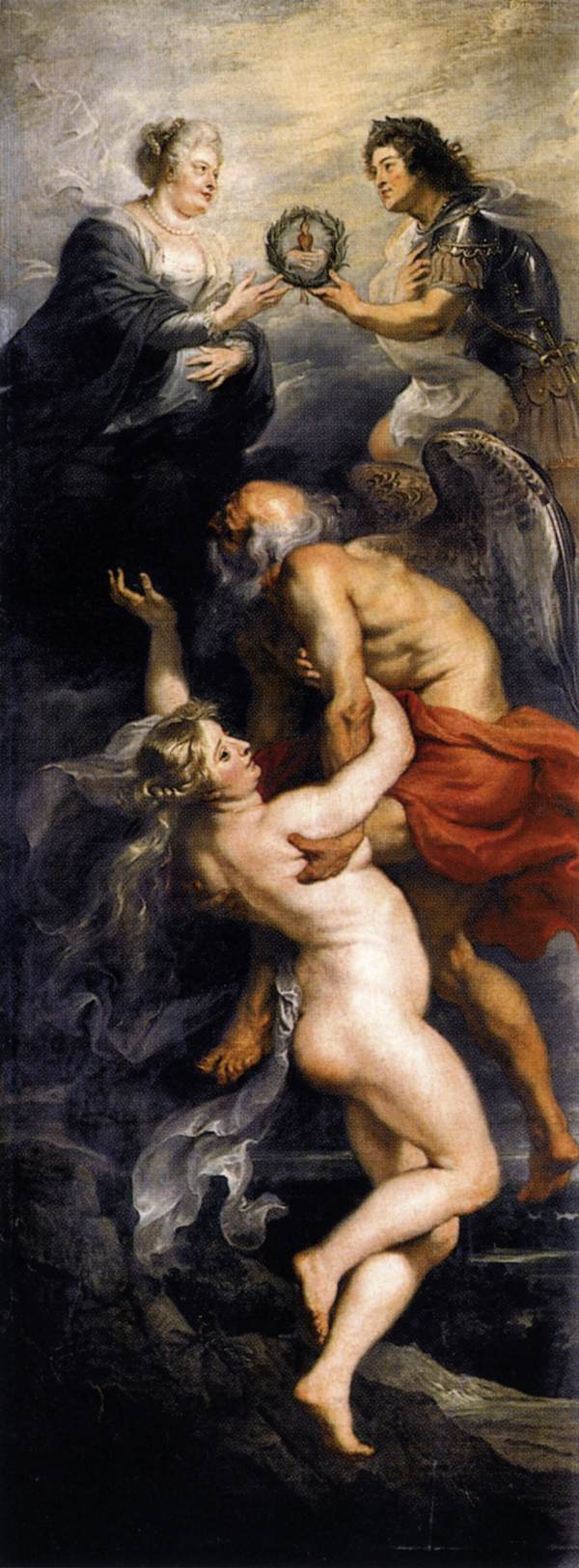In this tall, rectangular Renaissance-style painting, the scene is set against a gradient background that transitions from a dark black at the bottom to a light gray and white at the top. The focal point unveils four central figures in a vertical arrangement, embodying a rich tableau of human and divine interplay.

At the bottom stands a nude woman with light peach skin and long brown hair, her side facing the viewer, partly obscured by a muscular, older man with dark skin, grayish-white hair, and a matching beard. He sports angel wings and is clad only in a red garment draped around his waist, his left hand securely holding the woman's arm, stabilizing her on a rock-like platform.

Above them, two women, each elegantly robed in flowing, billowy garments, converge. The woman on the left dons armor over her outfit, combined with a dark cape, while her counterpart on the right, in a pure white robe with darker undertones, mirrors her posture. They both extend their hands towards each other, united in holding a wreath with a red candle at its center, positioned symbolically at the pinnacle of this vertical composition.

The absence of text within the image, the combined use of vibrant reds, soft grays, and stark whites, and the meticulous detailing suggest a painting not just of an era long past, but possibly of religious significance, underscored by the presence of angelic figures and the symbolic wreath and candle.